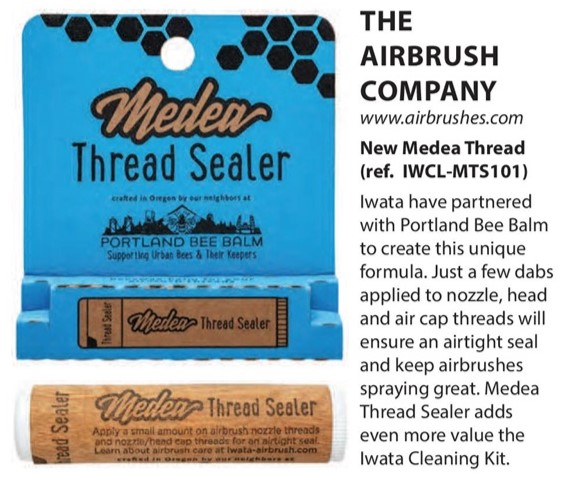The image depicts a detailed promotional layout for the Thread Sealer product by Portland Bee Balm. On the left half of the image, there are two pictures. The top picture features the product's cover, which is blue and displays the text "Media, Thread Sealer, Portland Bee Balm – Supporting Urban Bees and Their Keepers." The cover includes a black honeycomb design at the top and the text is in a combination of script and block lettering. Beneath this cover image, an illustration of the actual product is shown. The product resembles a cylindrical chapstick or lip balm, with a white body and a brown label that reads "Media Thread Sealer."

On the right side of the image, there is text in white against a black background. This text provides additional product information and reads: "The Airbrush Company, www.airbrushes.com. New Media Thread Sealer. Iwata have partnered with Portland Bee Balm to create this unique formula. Just a few dabs applied to nozzle, head, and air cap threads will ensure an airtight seal and keep airbrushes spraying great. Media Thread Sealer adds even more value to the Iwata Cleaning Kit."

Overall, the image combines graphical elements and textual information to highlight the functionality and collaborative creation of the product.